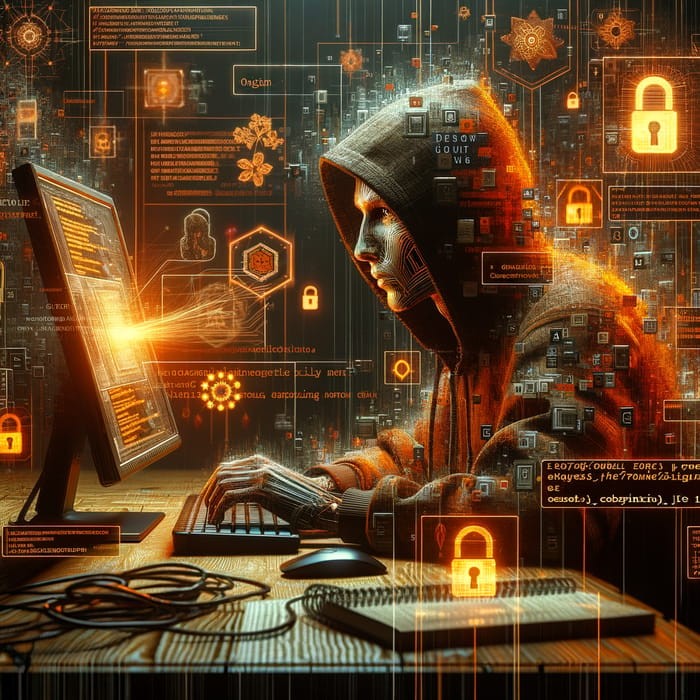A highly detailed and immersive digital or AI-generated artwork depicting a figure in a dark hoodie, characterized by its enigmatic and androgynous appearance. The figure's gray, illuminated skin features intricate orange highlights around the eyes and mouth, suggesting the presence of artificial lighting, possibly emanating from a computer screen. Technology-inspired patterns adorn their face, while their left hand has a mechanical aspect, hinting at a fusion between human and machine. 

The hood of the dark hoodie is pulled up, with drawstrings hanging down over the chest, and the sleeves taper at the wrists. The person is engaged in typing on a low-profile keyboard placed on a wooden desk. The computer screen displays a striking interface with a black background and vibrant orange text. A prominent gray square at the screen's center emits a bright orange light, illuminating the user. 

On the desk, a spiral notebook and a coiled wire add to the scene's authenticity, along with a flat mouse. The figure gazes intently at the LED screen that showcases various digital elements: lock symbols, pentagon shapes, and floral patterns, all representing a complex, digital information landscape in the dimly lit background, enhancing the futuristic and cybernetic ambiance of the artwork.